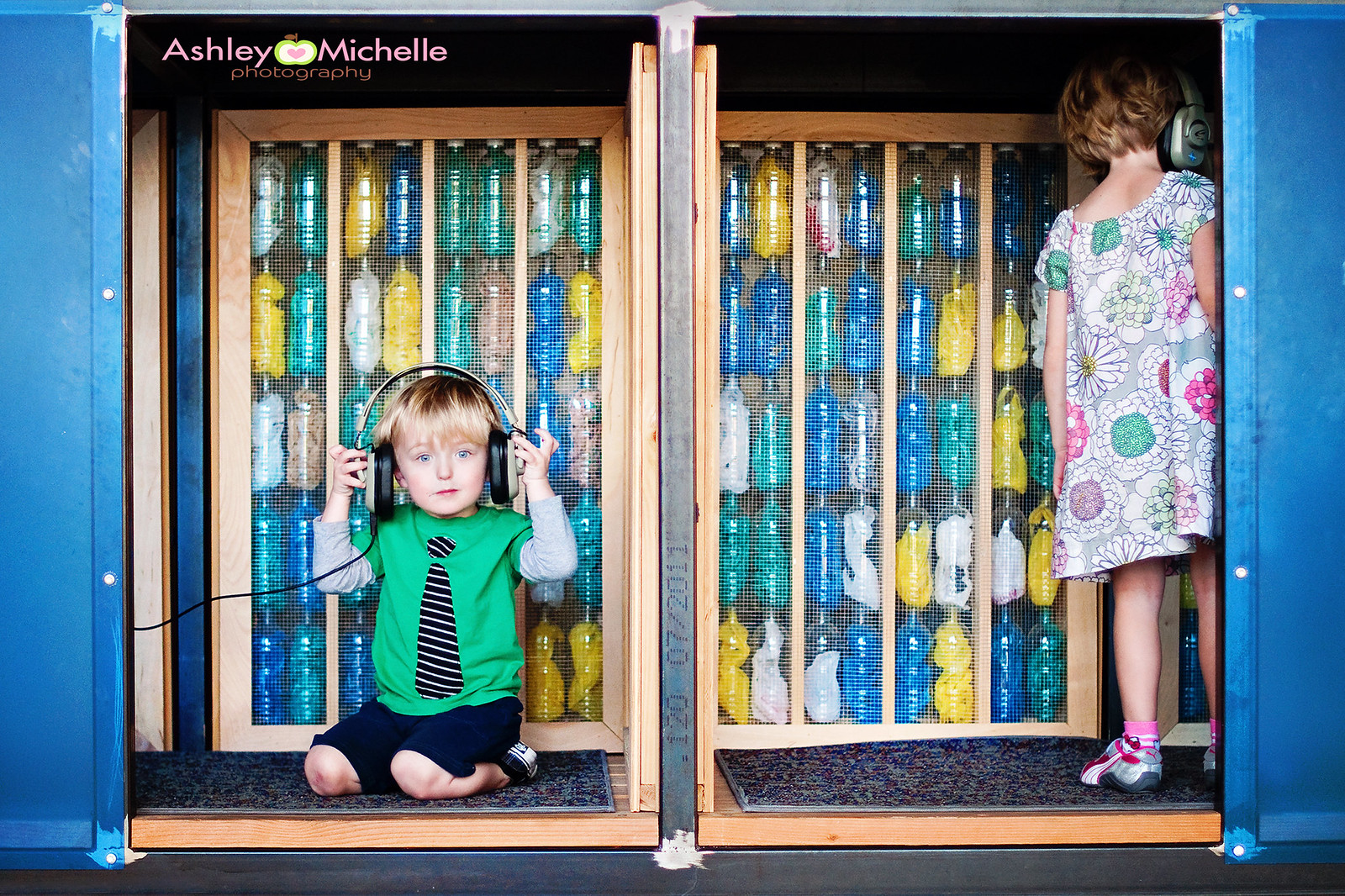In this vibrant, full-color photograph, two children are captured in a cozy indoor setting. On the left-hand side, a young blonde boy with blue eyes faces the camera. He kneels comfortably in a small alcove with a piece of black carpet, wearing a green short-sleeve shirt with a black and white striped tie graphic over a gray long-sleeve shirt, and blue shorts. The boy wears headphones, suggesting he's listening to music. Beside him, the alcove holds a shelf displaying colorful bottles in blue, green, white, and yellow hues.

To the right, a girl stands with her back to the camera, seemingly also in an alcove with a black carpet base. She has short hair and is dressed in a vibrant floral dress paired with pink socks, wearing headphones like the boy, and gazes towards the shelf of colorful bottles. The scene is set against a blue wall, adding a lively background to the image.

Above, text reads "Ashley Michelle" in pink, flanked by a heart-shaped apple core illustration, with "photography" written in smaller orange font below, indicating a touch of artistic branding in the snapshot.